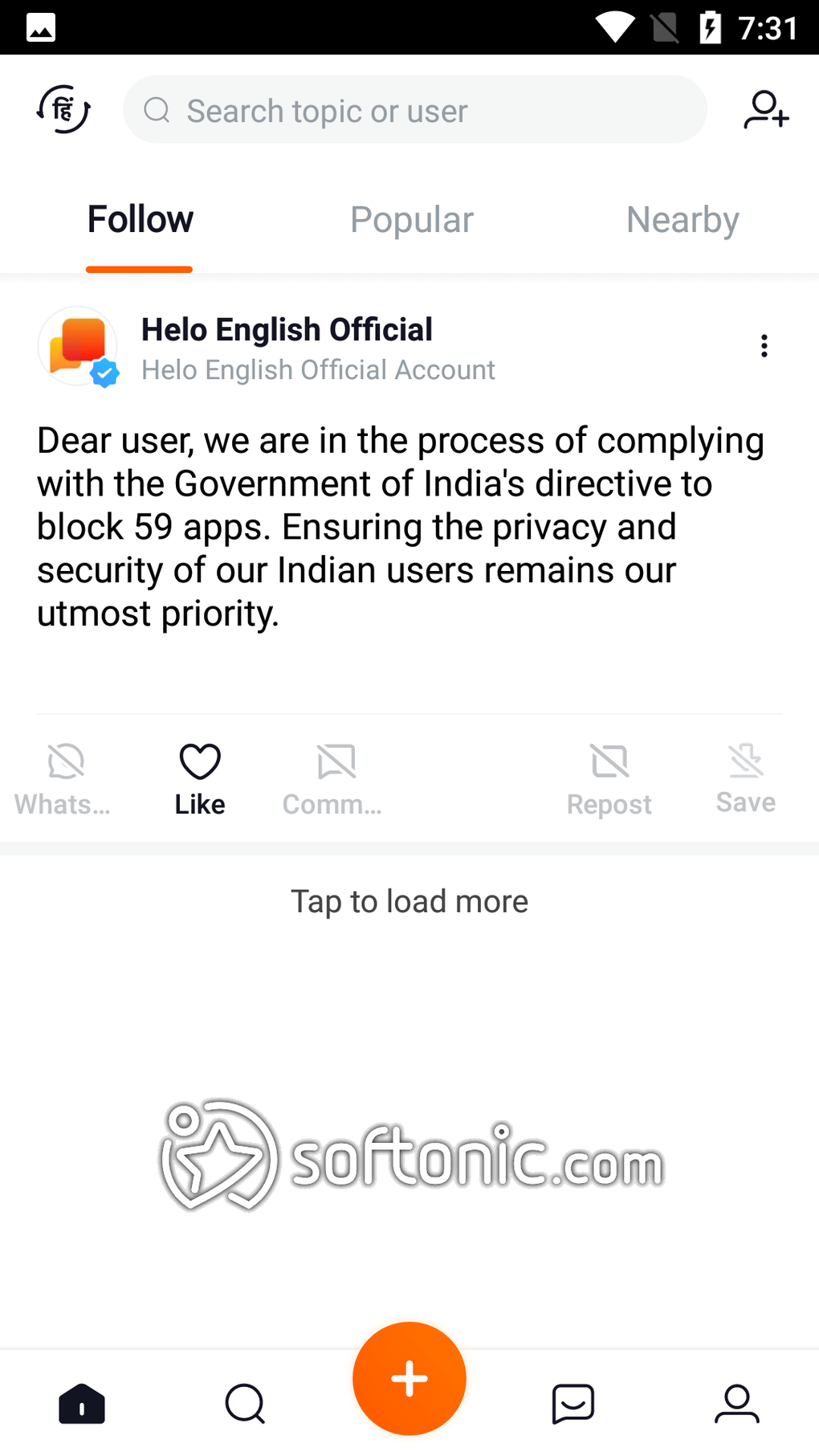**Descriptive Caption:**

A detailed screenshot of a mobile app interface is displayed. A watermark featuring a circle with a star and the text "softonic.com" is faintly visible. At the very top, the status bar shows an images icon, Wi-Fi signal, and a battery icon with a charging bolt, alongside the current time "7:31" in the right corner.

Just below the status bar is a search bar with the placeholder text "Search topic or user" and a profile/ad icon on the right side. Directly beneath the search bar are three selectable options: "Follow," "Popular," and "Nearby," with "Follow" highlighted.

The main section features a post from a user named "H-E-L-O English Official," with an orange speech bubble icon and a blue verified checkmark next to it. The text in the post reads: "We are in the process of complying with the Government of India's directive to block 59 apps, ensuring the privacy and security of Indian users remains our utmost priority."

Below the post are interactive buttons: a black "Like" button, and gray buttons for "Repost," "Share," and "Comment." At the bottom of the screen, there is an option to "Tap to load more" content. The app's footer features navigation icons for Home, Search, a Plus sign, and Profile.